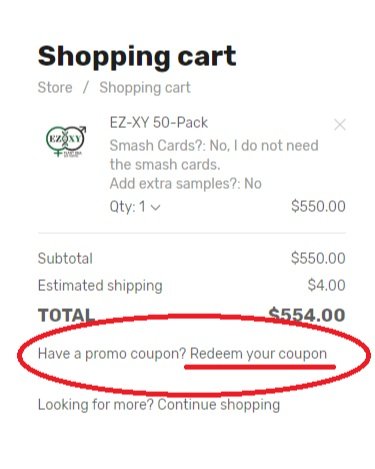### Detailed Caption:
The image depicts an online shopping cart's checkout page with a clean white background. At the top left, the text "Checkout" is displayed in black. Directly below, in bold black font, "Shopping Cart" is written with a capital "S". Beneath this, "Store / Shopping cart" is listed in light gray, with "Shopping" capitalized but not "cart".

The selected item is an "EZ-XY 50-pack". The item's icon, displayed to the left, consists of the male and female symbols: a circle with an arrow pointing up and to the right, and another circle with a cross pointing down. These symbols are interconnected, and the letters "EZ-XY" are inscribed within the conjoined circles.

Directly under the item name, "EZ-XY 50-pack", the text "Smash Cards" appears in light gray. This is followed by the options "No, I do not need the Smash Cards." and "Add extra samples? No." The quantity selected for the item is one. A light gray 'X' appears in the top right corner next to the item's details.

To the right of the quantity, the price is displayed as $550. Below this section, a light gray line demarcates the pricing summary. Following this line, the text "Subtotal $550", "Estimated Shipping $4", and "Total $554" are sequentially listed.

Further below, the section inviting the use of discounts says, "Have a Promo Coupon? Redeem Your Coupon." Just beneath this, the page offers a link, "Looking for More? Continue Shopping." The phrase "Have a Promo Coupon? Redeem Your Coupon" is encircled in red, and the words "Redeem Your Coupon" are further underlined in red for emphasis.